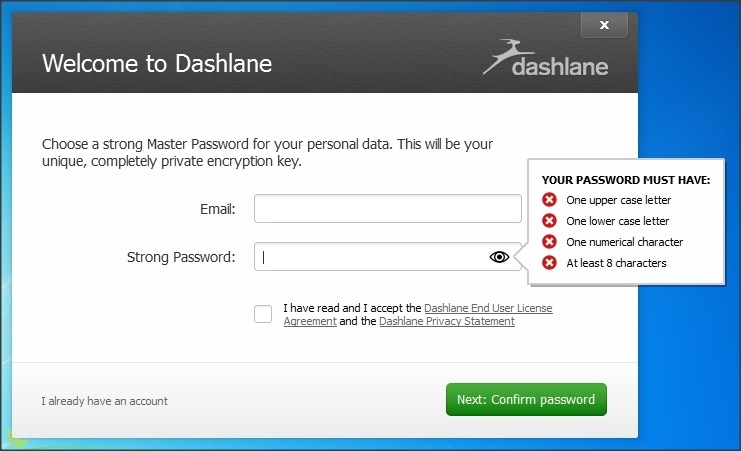The image is a screenshot of a computer screen displaying an open window with a blue background. The website currently open is Dashlane, indicated by a welcome message in white text on a charcoal gray background. On the right-hand side of the window, a deer is depicted in a leaping pose, jumping diagonally from the seven o'clock position to the one o'clock position. Underneath the deer's extended legs, the word "Dashlane" is written in lowercase letters.

The main portion of the image features a white background with instructional text that reads, "Choose a strong master password for your personal data. This will be your unique, completely private encryption key." Below this message is a blank, rectangular text field labeled "email:" on the left side. Another blank text field labeled "strong password:" is situated below the email field, with an eyeball symbol on its right side. To the right of this symbol is a gray-outlined box containing bold black text that instructs, "Your password must have:".

Within this box, four red circles with white Xs precede the following requirements: one uppercase letter, one lowercase letter, one numerical character, and a minimum of eight characters. Below the password guidelines is a toggle box with text stating, "I have read and accept the Dashlane end user license agreement," and "Dashlane privacy statement," both of which appear to be hyperlinked.

At the bottom left of the window, there is a highlighted option stating, "I already have an account." On the bottom right is a rectangular green button with white text that says, "Next confirm password."